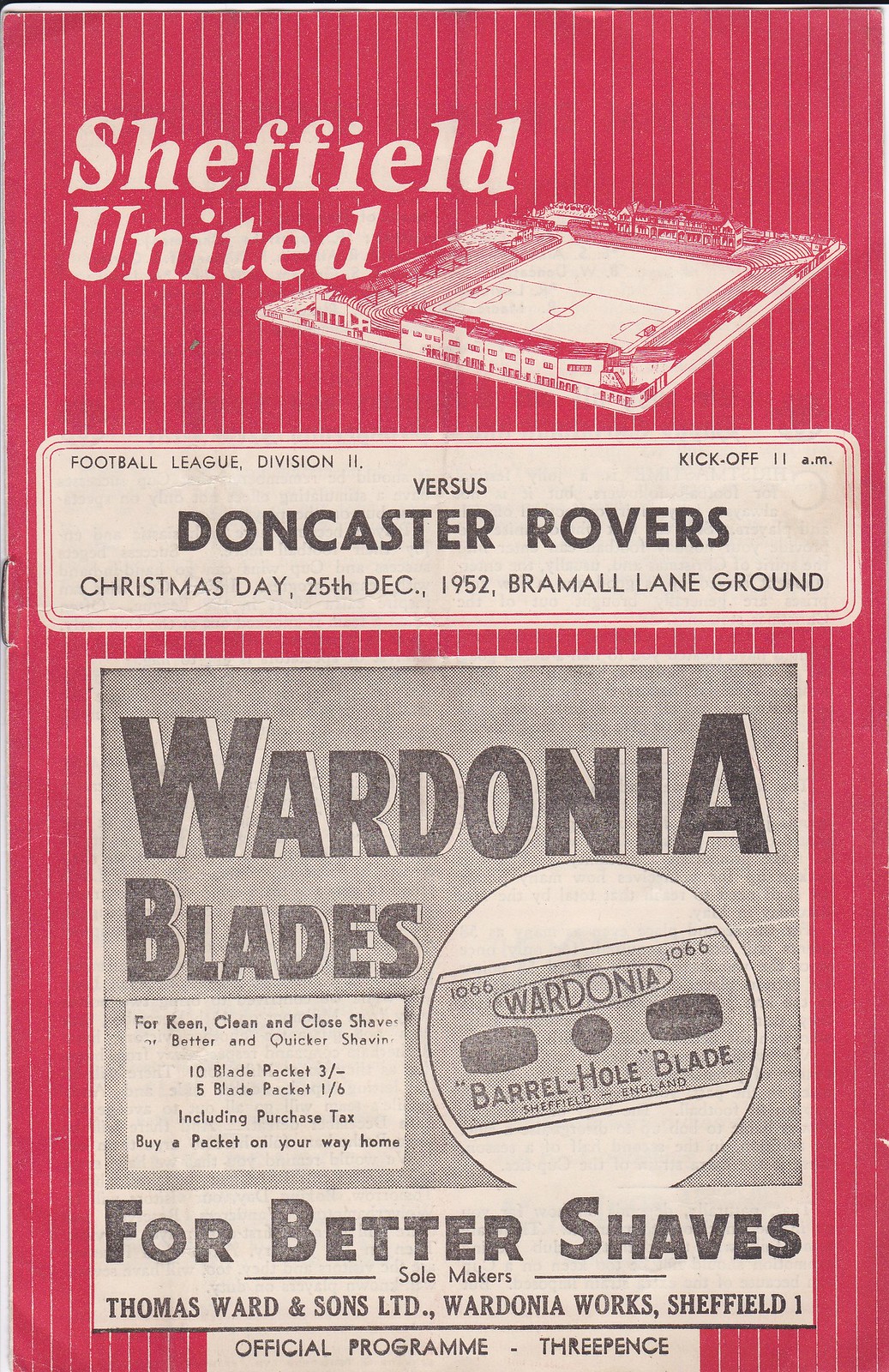The image is a vintage advertisement from a 1952 Sheffield United football (soccer) match against Doncaster Rovers, printed on a portrait-oriented flyer with a red background and white vertical pinstripes. At the top, bold italic serif text reads "Sheffield United" next to an angled image of a soccer field at Bramall Lane Ground, equipped with stadium seating and two mansion-like structures at either end. The flyer details include "Football League Division Two" and "versus Doncaster Rovers, Christmas Day, 25th December 1952," with a kickoff time of 11 a.m. Below this, a black and white ad for Wardonia Blades occupies the bottom half, promoting "keen, clean, and class shaves" with an image of the blade and the slogan "For better shaves." The flyer is marked as the "official program" and priced at three pence. The overall style reflects vintage printing techniques, indicative of an era gone by.